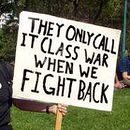The image is a very small, rectangular, and low-quality picture, almost like a thumbnail. It features a scene set outdoors in a grassy field with darker green trees in the background, and a light blue sky visible on the left side. The main focus is on a person with white skin, wearing a black T-shirt, holding a white picket sign with big black text that reads: "THEY ONLY CALL IT CLASS WAR WHEN WE FIGHT BACK." The handle of the sign is wooden. To the right side of the photo, a green pole can be seen, and partially visible is another person sitting in the grass, identifiable by a blue sleeve and a white-skinned hand. There is also a faint image that might be a swing set in the background.